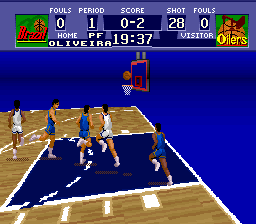The screenshot captures an older, pixelated basketball video game. At the top of the image, the scoreboard displays that Team Brazil, in red text, is playing the Oilers, in yellow text with an overlay of a basketball and oil drill. The scoreboard details include: Brazil listed at the upper left with 0 fouls, period 1, and 0 points, while the Oilers, listed at the upper right, show with 28 shots, 0 fouls, and 2 points. The home and visitor indicators are also present, with the time set at 1937. The basketball court features a blue background on the walls, a tan floor with white lines, and a blue free-throw area. The basket has a white net and an orange backboard. On the court, five players are visible: three in blue jerseys and shorts, and two in white jerseys and shorts. A basketball hovers just above the net, indicating an active play.